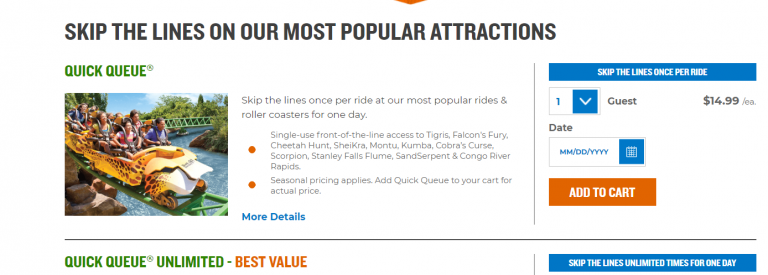The image is a screenshot of a theme park's online booking system, which offers different types of "skip the line" passes for its most popular rides and roller coasters. The page advertises various options, including the "Quick Way" pass that allows visitors to skip the line once per day for each ride, and the "Quick Way Unlimited Best Value" pass, which offers unlimited skips for a single day. 

Specific rides mentioned include Falcon's Fury and Cheetah Hunt, though the exact theme park is not identified in the screenshot. Visitors can choose the number of guests, the date of their visit, and add the selected pass to their cart. The system appears to charge $4.99 per person for the passes. The layout includes clickable buttons for selecting the "Quick Way" or the "Quick Way Unlimited Best Value" options, facilitating an easy purchase process for those looking to maximize their ride experience by avoiding long lines.